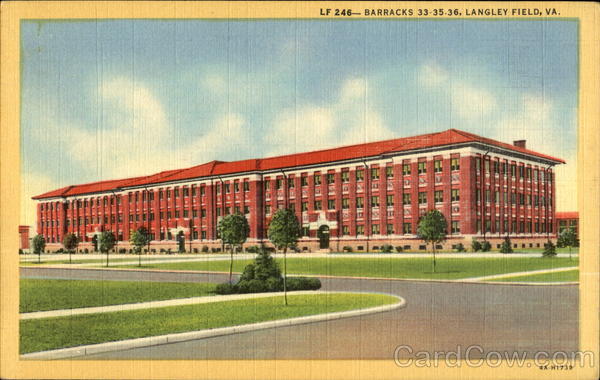This image is an artistic illustration resembling an old postcard, depicting the barracks 33, 35, and 36 at Langley Field, Virginia. The building is a long, wide, rectangular structure, approximately three to four stories high. It features numerous regularly spaced windows across its red brick facade, complemented by a vibrant red angled roof. Positioned on a meticulously manicured lawn, the scene includes evenly spaced, small trees with thin trunks and some bushes at the base of the building. The front of the barracks faces a gray street bordered by areas of green lawn and intersected by gray sidewalks. The sky above is a light blue adorned with wispy white clouds. Encircling the image is a yellow-beige border, with text in the upper right corner reading "LF246, Barracks 33, 35, 36, Langley Field, Virginia." Additionally, there is a faint website URL, cardcow.com, at the bottom right of the border. The composition has a nostalgic, uniform, and serene military base ambiance, with no visible human activity or vehicles on the street.